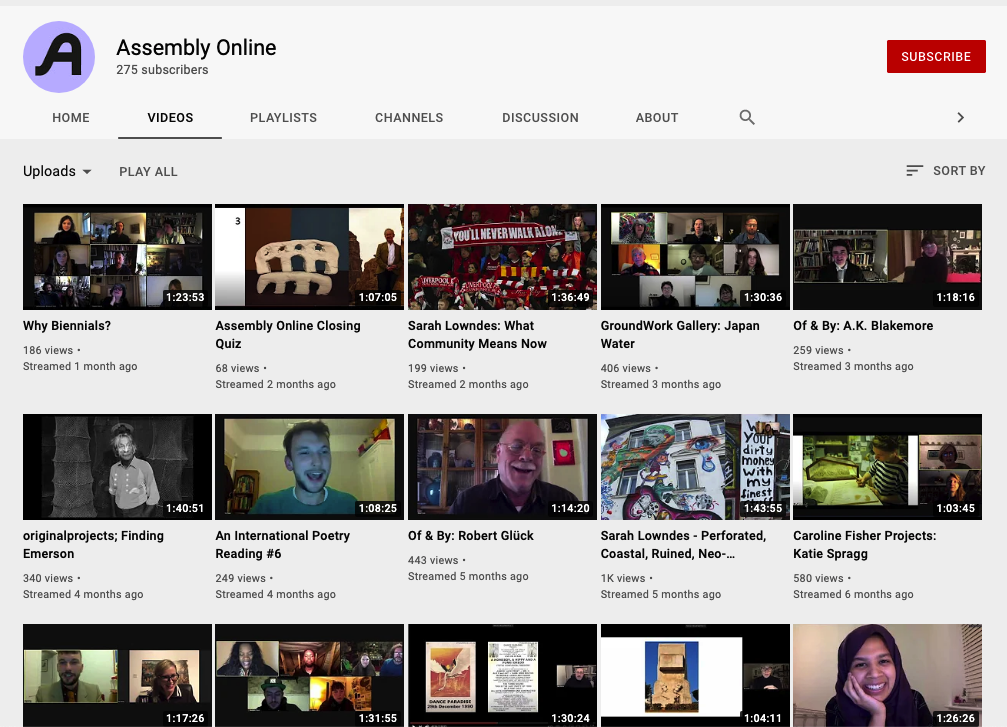**Descriptive Caption:**

Screenshot of the "Assembly Online" YouTube channel, showcasing a snapshot of its videos and subscriber count. The channel, which has 275 subscribers, features an icon with a black "A" inside a purple circle. 

The video section is organized into three rows, each containing five videos, making a total of 15 visible uploads. The videos encompass a range of topics, including live streams, project showcases, and interviews. Here's a detailed list of the videos starting from the top-left:

1. **"Why Biennials?"**  
   - 186 views
   - Streamed one month ago

2. **"Assembly Online Closing Quiz"**  
   - 68 views
   - Streamed two months ago

3. **"Sarah Lounge: What Community Means Now?"**  
   - 199 views
   - Streamed two months ago

4. **"Groundwork Gallery: Japan Water"**  
   - 406 views
   - Streamed three months ago

5. **"OFNB: Cape Lake"**  
   - Views not specified

6. **"Original Projects: Finding Emerson - An International Poetry Reading"**
   - Not included in the initial description, hence views not specified

7. **"Overn by Robert Gluck"**
   - Not included in the initial description, hence views not specified

8. **"Sarah Lounge: Perforated Coastal Ruin"**
   - Not included in the initial description, hence views not specified

9. **"Neo Carolyn Fisher Projects: Katie Sprague"**
   - Not included in the initial description, hence views not specified

The bottom row contains five videos that are partially cut off, displaying a mixture of Zoom calls, artistic events, and project discussions. This rich variety of content provides a glimpse into the engaging and diverse offerings of the "Assembly Online" channel.